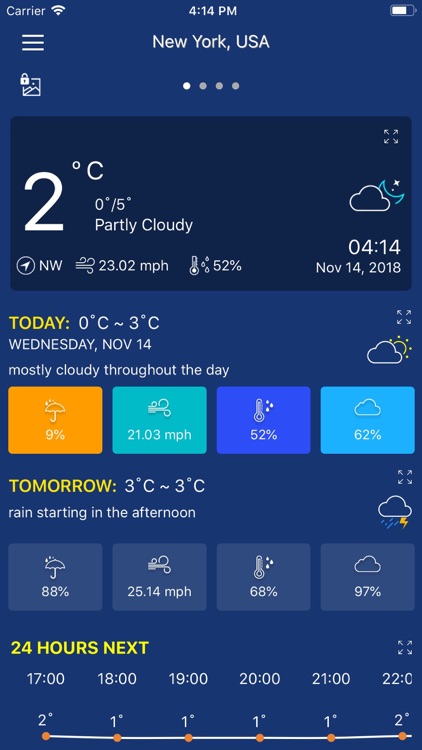In the image, a smartphone screen displays a weather application, with intricate details starting from the top of the screen. At the top, there is a series of icons, including the cellular carrier signal, the Wi-Fi signal, the current time displayed as 4:14 PM, and the battery life indicator. Below these icons is a menu button. Centered on the screen is the location "New York, USA," and beneath it, there are four dots indicating the number of pages within the app, with the first dot highlighted in white.

Directly below, a box displays the current temperature in New York, flanked by today's forecasted temperature range. The current date is listed underneath. Following this, a textual description reads "Mostly cloudy throughout the day," accompanied by an icon representing cloudy weather on the right. Further down, there are four distinct color-coded boxes: 

1. An orange box indicating precipitation levels.
2. A light blue (more greenish) box representing wind gusts.
3. A dark blue box showing the current temperature.
4. Another light blue box displaying the cloud status.

Below these boxes, the app shows tomorrow's weather forecast and temperature range. Finally, at the bottom of the screen, there is a detailed 24-hour forecast summary. The composition delivers a comprehensive overview of the weather conditions and forecasts in New York.